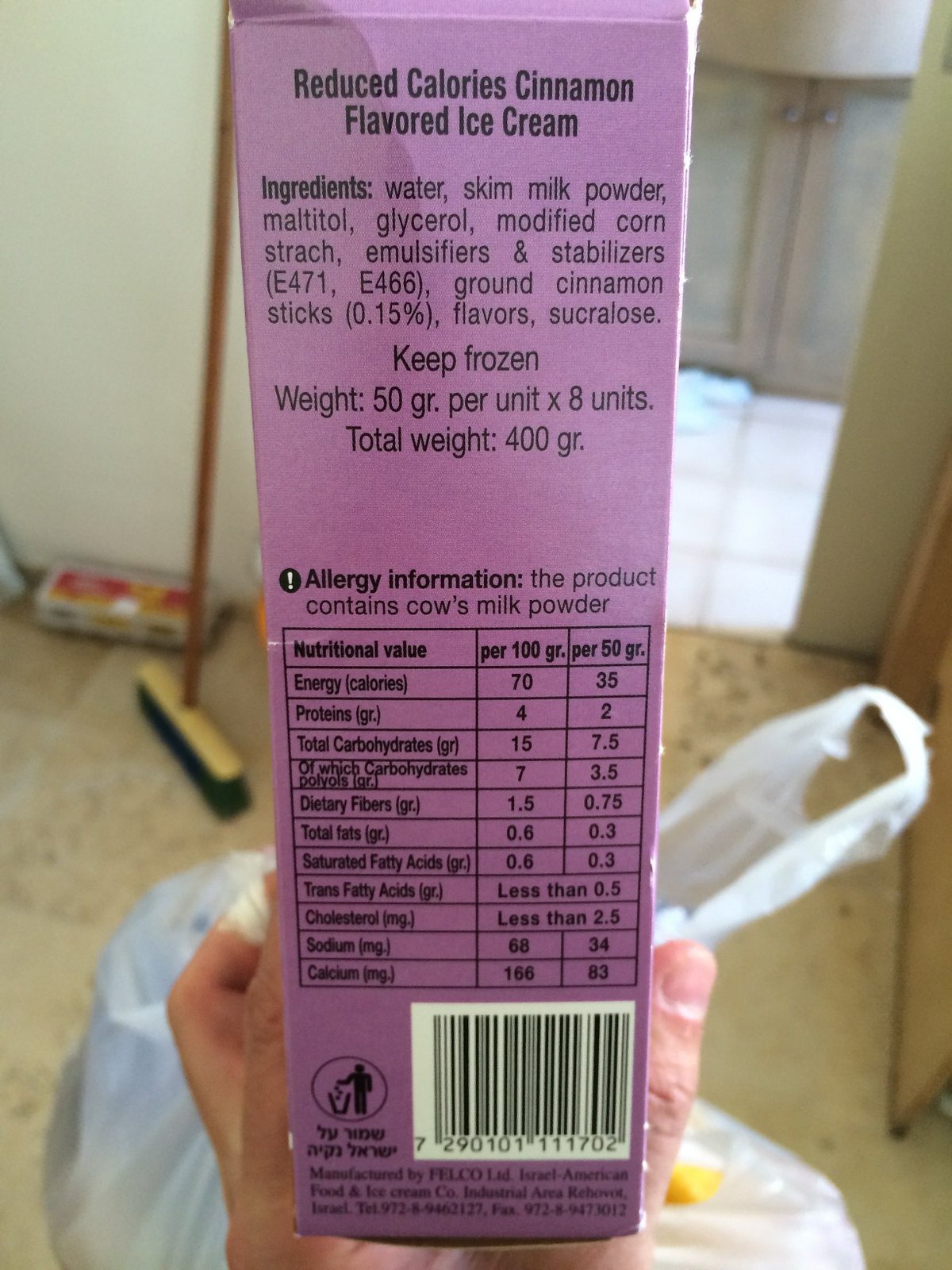This detailed color photograph captures a close-up view of a food or drinks carton, held by a person's hand, visible at the bottom of the frame and slightly out of focus. The perspective suggests that the viewer is looking down at the scene from above. The carton itself is predominantly a purple-pink hue, with a white barcode located at the bottom right.

The carton prominently features black text. At the top, it reads "Reduced-Calorie Cinnamon-Flavoured Ice Cream." Beneath that, an ingredients list is displayed along with storage instructions advising to keep the product frozen. The carton specifies that each unit weighs 50g with a total package weight of 400g across 8 units. It also includes allergy information and a detailed nutritional table listing energy, protein, total carbohydrates, cholesterol, fat, and other relevant data. In the lower left-hand corner, there is a small logo depicting a person disposing of the carton in a recycling bin, emphasizing proper disposal to avoid littering.

The background includes a white bag, which appears to contain a yellow object, positioned just under the person's hand. On the left side of the image, a wooden floor is adorned with a sweeping brush that has a long, thin wooden handle. Adjacent to a grey wall, a red and white box can also be seen. Towards the right side, there is a doorway leading into another room, which has light, almost white, tiles on the floor. A greyish cupboard with a round object on top, likely a sink, is visible within this adjoining space.